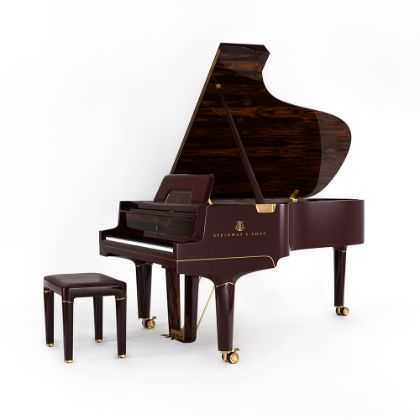The photograph displays a dark mahogany grand piano and matching stool set against a clean, white backdrop. The piano's top lid is propped open, revealing the dark wood interior, and the cover over the keys is raised, displaying the white and black keys as if awaiting a tuning session. The piano is equipped with gold wheels for easy movement, and golden accents highlight various features such as the ends of the piano bench legs, pedals, and small decorative stripes along the body, though the writing on the body is illegible. The scene captures the timeless elegance of the piano with no sheet music or people present, emphasizing its solitary grandeur.